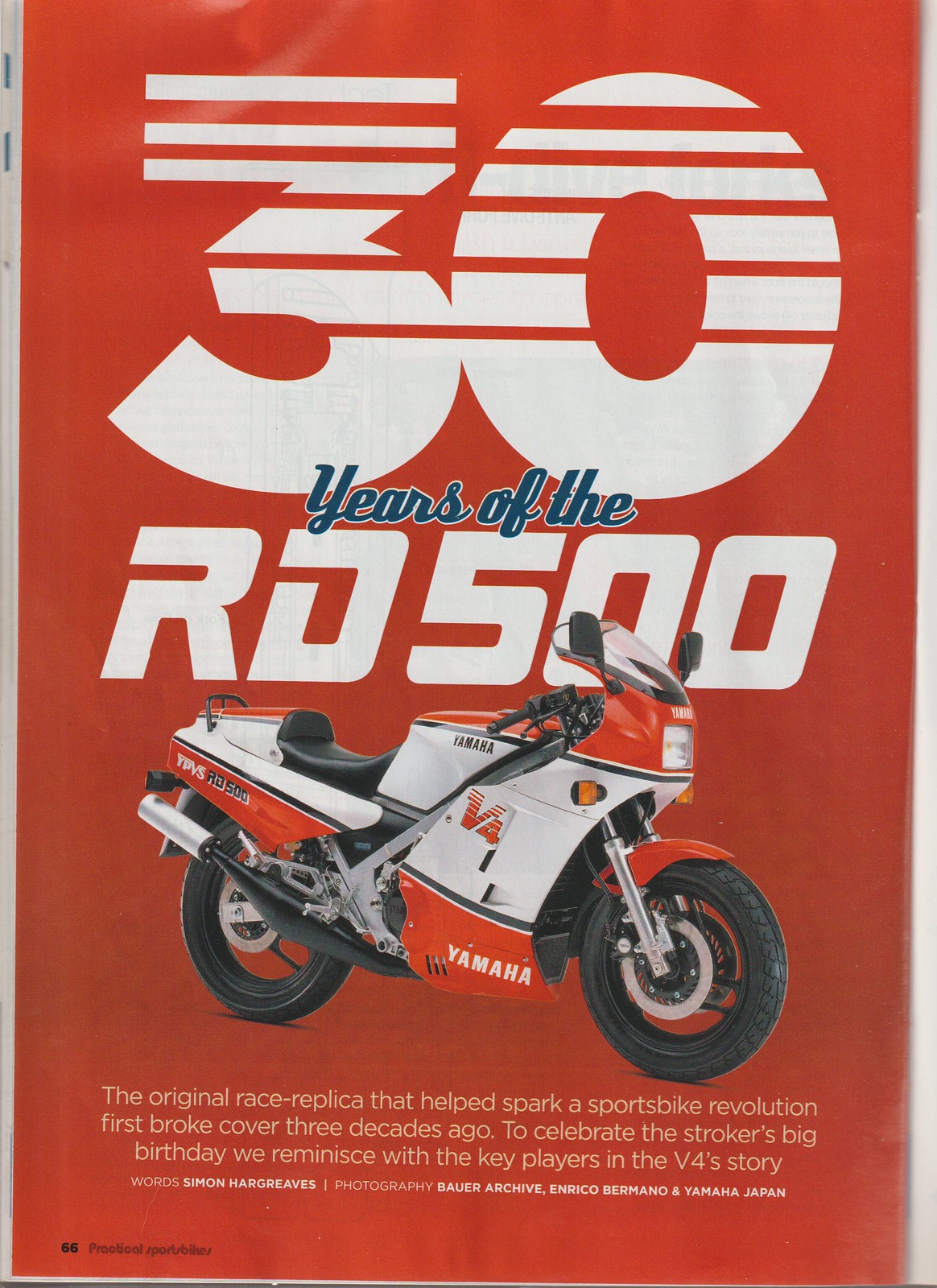The magazine page features a vibrant advertisement for Yamaha, celebrating "30 years of the RD500." Dominated by a striking red background, the page has prominent white text, with the number "30" in large print, accompanied by blue text reading "years of the." Beneath this, the text continues with "RD500," showcasing a sporty motorcycle directly below. This motorcycle has a distinctive color scheme: red on the bottom and top parts of the frame, with a white middle section, extending up to a small windshield. The bold Yamaha logo is displayed at the bottom of the motorcycle. The accompanying caption highlights the significance of the RD500, noting it as "the original race replica that helped spark a sports bike revolution" when it was introduced three decades ago. The text also mentions that to celebrate the milestone, the ad reminisces with key figures in the V4 story. Photographers and contributors such as Simon Hargreaves, Bear Archive, Enrico Romano, and Yamaha Jim are credited for their work in the ad, which nostalgically honors this revolutionary bike's history.